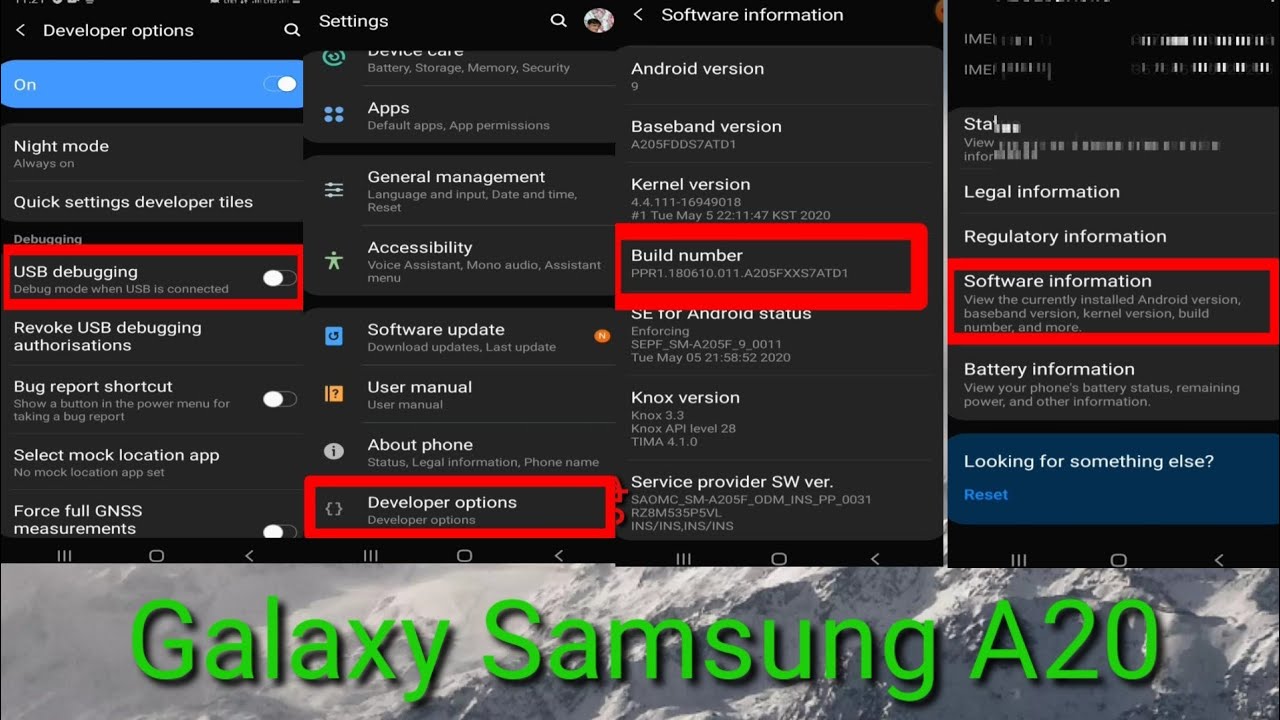This image is a detailed instructional screenshot for troubleshooting or configuring settings on a Samsung Galaxy A20. The bottom half of the screen features a serene background of snow-capped mountains, over which the model name "Galaxy Samsung A20" is displayed in a vibrant green text with a shadow effect. Above this, the top half showcases four vertical screenshots of the phone's Android operating system, specifically focusing on the settings menu.

The screenshots, set against a predominantly gray background with white text, highlight key areas within the developer settings. Each screenshot has red highlighted sections to draw attention to specific options:

1. The first screenshot emphasizes "USB debugging."
2. The second highlights "Developer options."
3. The third marks "Build number."
4. The fourth points out "Software information."

These highlighted sections are likely intended to guide users through important steps or settings adjustments on their Galaxy A20, providing a visual aid for resolving issues or enabling developer features efficiently.